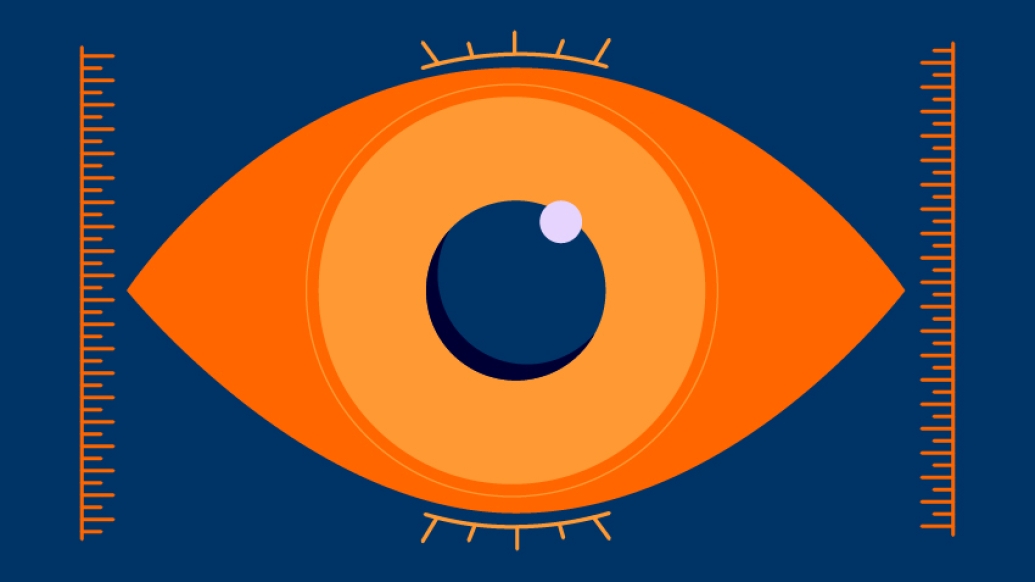This is a digital art image featuring a prominent, stylized eye set against a dark navy blue rectangular background. The eye itself is football-shaped with an outer area in vibrant orange. Inside the eye, there is a paler orange concentric circle forming the iris, and at its heart is a dark blue pupil. The pupil includes a small white circle towards the top right, giving it a reflective, 3D effect. Bordering the eye on the left and right are vertical orange lines with fine horizontal dashes, reminiscent of millimeter markings on a ruler. Above and below the eye are slightly curved, spaced-out lines in a lighter orange shade, suggesting an eyelash effect. These lines are similar to the ones flanking the eye, but they are fewer and more widely spaced, contributing to an intricate and balanced composition. Despite the detailed elements, the overall context of the image remains abstract.